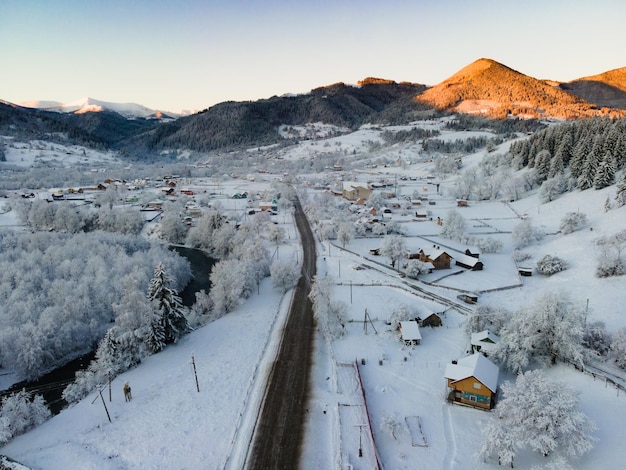In this breathtaking overhead shot, the serene winter landscape unveils a small, picturesque community nestled in a valley beneath a clear, pale blue sky, devoid of clouds. The sun casts a soft, golden glow over the scene, illuminating the snow-covered ground, trees, and bushes that dot the landscape. A contrasting range of mountains frames the background: the furthest peak is capped with snow, transitioning to dirt-covered and then blue ridge mountains as they draw closer. 

A winding asphalt highway and a set of rail tracks thread through the town, which is divided by scattered and increasingly dense houses on either side. The road leads up towards the mountains, bordered by fenced fields and marked by the occasional power pole. To the left of the main road, there is a cluster of five or six houses, hinting at a close-knit community. The valley is full of life with intermittent greenery. The entire scene is viewed from a high vantage point, likely captured by a drone, offering a panoramic perspective that highlights the tranquil, snowy expanse and the intricate layout of this quaint village.